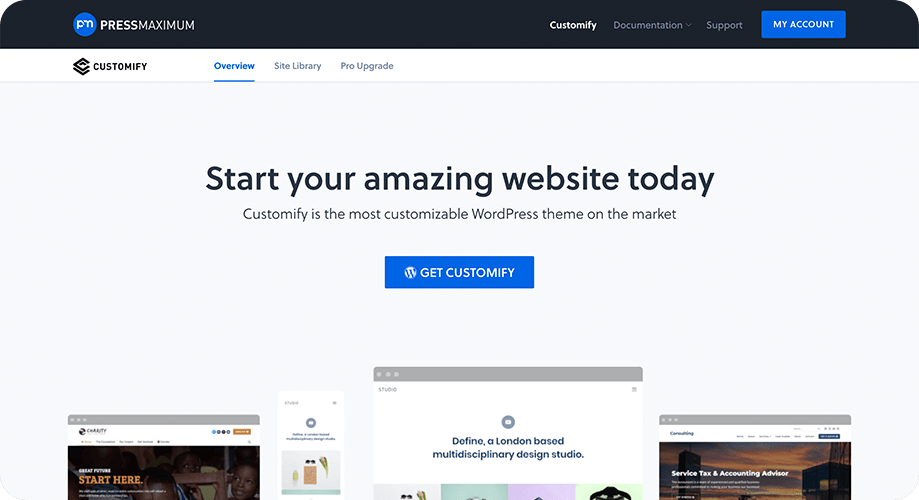In this detailed photograph of a webpage, the central focus is on an interface section featuring a circle icon with the letters "P" and "M" in white. Adjacent to it, the text "Press Maximum" is prominently displayed in white. To the right of this section, the phrase "Customify Documentation" appears alongside a downward pointing arrow indicating additional support options. A blue button labeled "My Account" is situated nearby.

The topmost part of the webpage, set against a clean white background, showcases the brand name "Customify" accompanied by a distinctive stacked diamond logo. The "Overview" tab is highlighted in blue, indicating it is the selected section, while the "Site Library" and "Pro Upgrade" tabs are presented in a subdued gray font.

The body of the page reads, "Start your amazing website today. Customify is the most customizable WordPress theme on the market." Below this encouraging call to action, there is a prominent blue button labeled "Customify". Toward the bottom of the page, there are multiple screen grabs displaying different website designs. These varied designs include a black and orange theme, a pink, green, and dark green theme, and one featuring a sky scene.